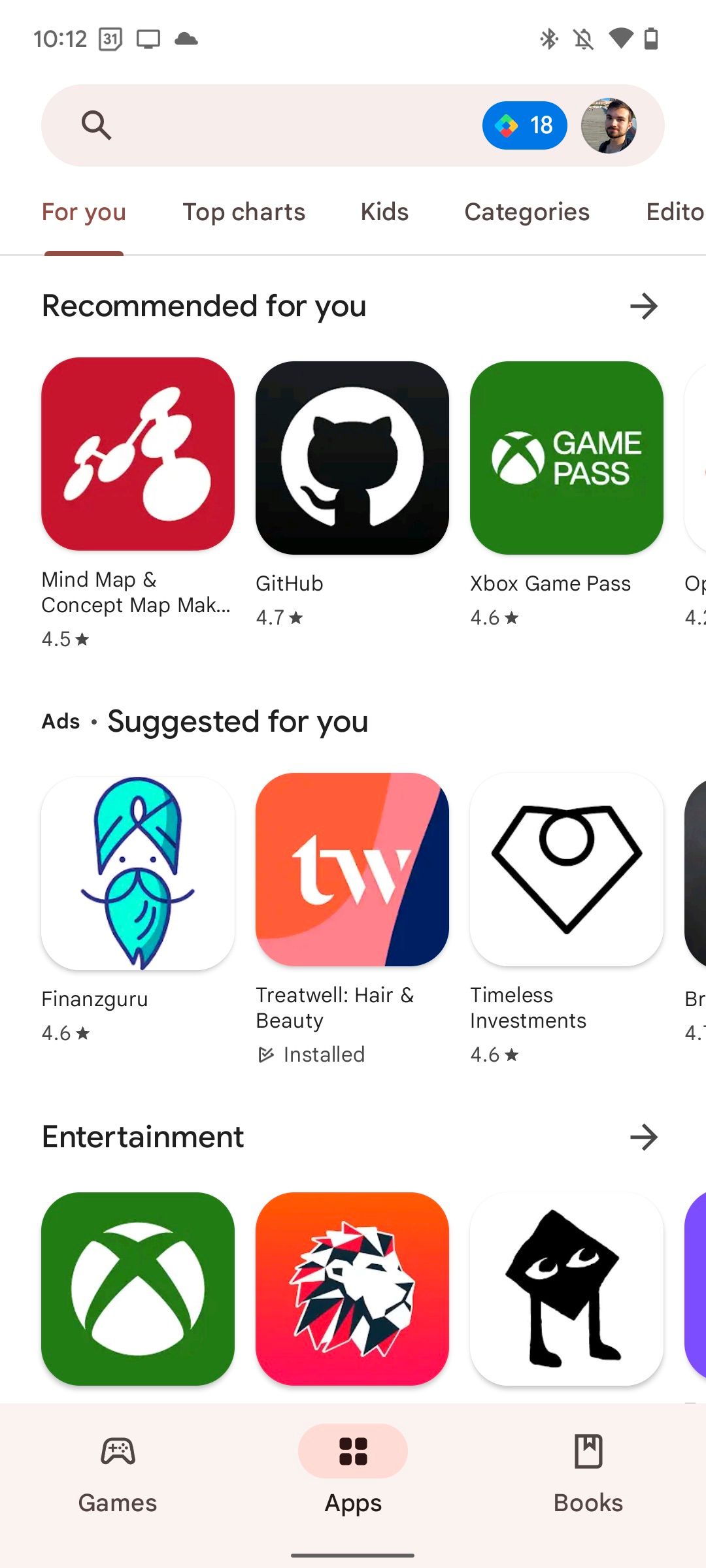Here is a cleaned-up and detailed caption for the described screenshot:

---

The screenshot displays a smartphone screen at 10:12 AM. The interface shows the notifications turned off, with Bluetooth enabled and a robust internet connection. The weather indicates cloudy conditions and the battery is running low. 

At the top of the screen, a search bar is visible, accompanied by the user profile icon. Below this, several tabs are listed: "For You" (highlighted in brown), "Top Charts," "Kids," "Categories," and "Edit," with the rest in gray. The current tab is "For You," displaying personalized content recommendations.

The first row under "Recommended for You" features apps like "Mind Map and Concept Map," "GitHub," identified by its logo, and "Game Pass." 

The following section titled "Ads: Suggested for You" includes "Finance Guru," "Treatwell" (a health and beauty app), and "Timeless Investments."

Under "Entertainment," "Xbox," an app with a lion icon, one unidentified app, and another app featuring a cube with feet are shown.

At the bottom of the screen, navigation options for "Games," "Apps," and "Books" are present, with the "Apps" section currently open.